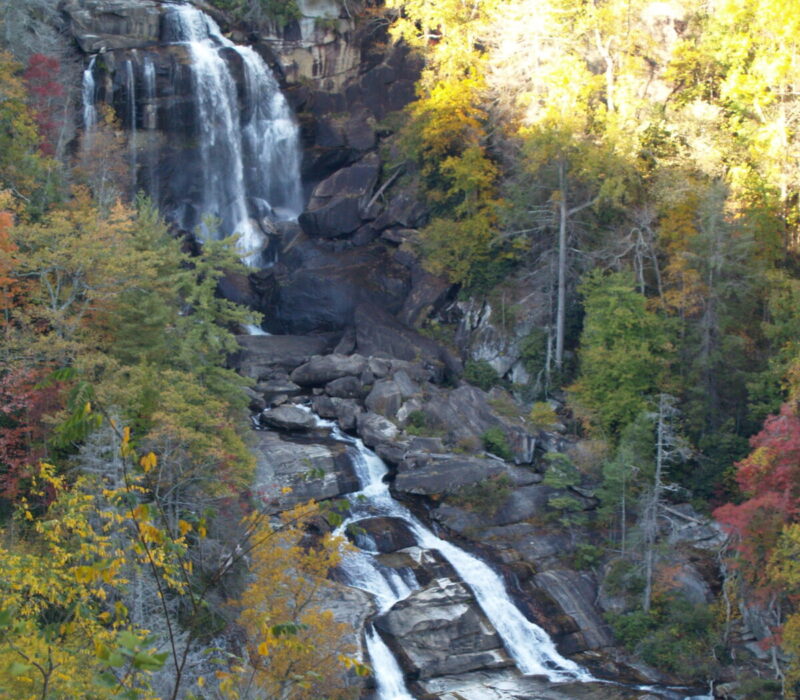This square-shaped, photorealistic (though somewhat low-definition) photograph captures a serene outdoor scene featuring a cascading waterfall amidst autumnal forest terrain. Dominating the upper left quadrant, the waterfall spills over dark brown and gray rocks in two main streams, accompanied by several smaller streams and mist. The water, white and lively, flows down the rocky ledge, weaving through large boulders and creating whitewater rapids as it advances towards the bottom right of the image.

The waterfall is flanked by lush trees, predominantly evergreens, punctuated with deciduous trees showcasing autumn hues of red, yellow, and green. The right side of the scene reveals more greenery interspersed with spots of yellow-leafed trees, suggestive of the season. The top right corner is bathed in bright sunlight, casting a golden glow on the upper foliage, while the majority of the landscape remains shadowed, accentuating the natural textures and muted colors.

Overall, this photograph beautifully captures the essence of a vibrant yet tranquil waterfall in an autumn forest, highlighting the interplay of rushing water and colorful foliage under dappled sunlight.